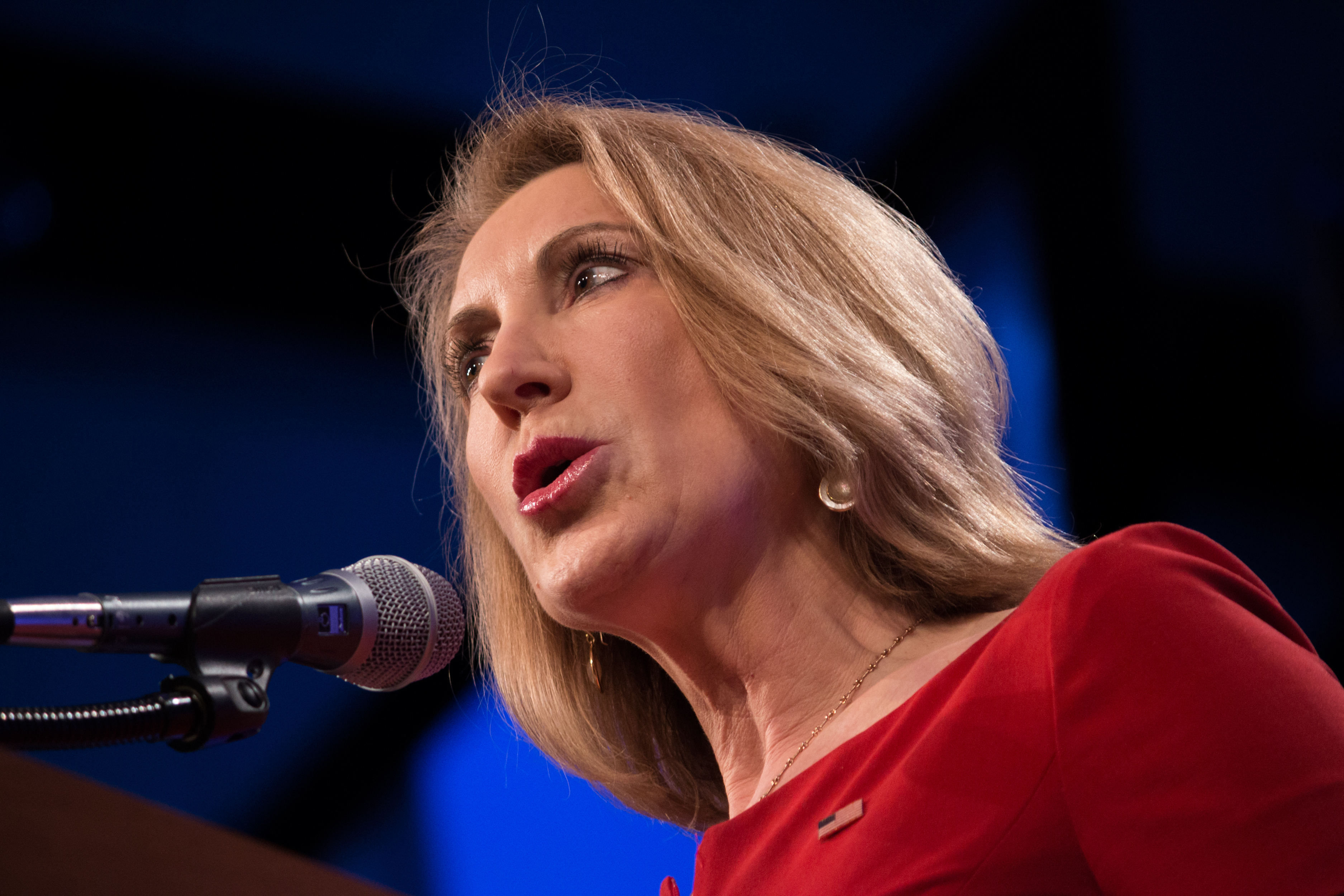The image features a close-up of a white woman with medium-length blonde hair and red lipstick, speaking into a microphone. Her angle is slightly upwards, and she appears to be looking off to her right, almost in profile. The microphone, which has a silver head and a black stand, is positioned to the left in the image. The woman is dressed in a red long-sleeve blouse, adorned with an American flag pin above her left breast. She also wears a thin gold chain necklace and round gold earrings. The background is primarily dark blue and black, with a lighter blue backlight highlighting her head, creating a contrast that makes her stand out. A brown podium is partially visible in the lower left corner.